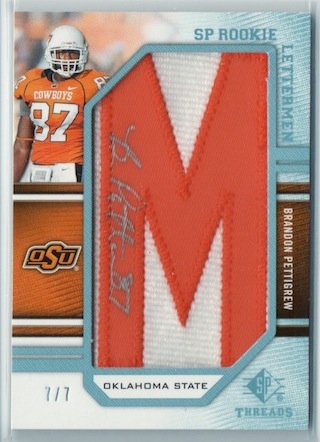This is a highly detailed sports trading card featuring football player Brandon Pettigrew. The card has a light blue border surrounding a central area dominated by a large, red, fabric letter "M" on a light tan or gray background. The "M" has distinctive diagonal cuts on the upper left and lower right parts, adding a unique design element. Encased within the "M" is a printed autograph, which adds to its collectible value. 

In the top left corner of the card, there is an inset photograph of Pettigrew in an orange jersey emblazoned with "Cowboys" and the number 87. He is wearing a white helmet, and the background behind him is a blurred outdoor scene. Adjacent to the upper right corner of the fabric M, the text "SP Rookie" is prominently displayed in dark blue. Vertically along the right side, in slightly lighter blue text, is the word "Letterman."

At the bottom of the "M" section is a white field with "Oklahoma State" written in dark blue. Below this, on the right side, is a vertical brown rectangle with white text displaying "Brandon Pettigrew." This is followed by another blue section featuring a diamond graphic and the word "Threads" in dark blue text.

On the left side, below the photograph, there is an orange vertical rectangle with white bars at the top and bottom containing the letters "O-S-U," with the "S" being larger and centrally positioned. Below this orange rectangle is a horizontal blue bar, and underneath that, the card indicates "7/7," which likely signifies its limited edition status. The entire card is protected in a clear plastic cover, emphasizing its collectible status.